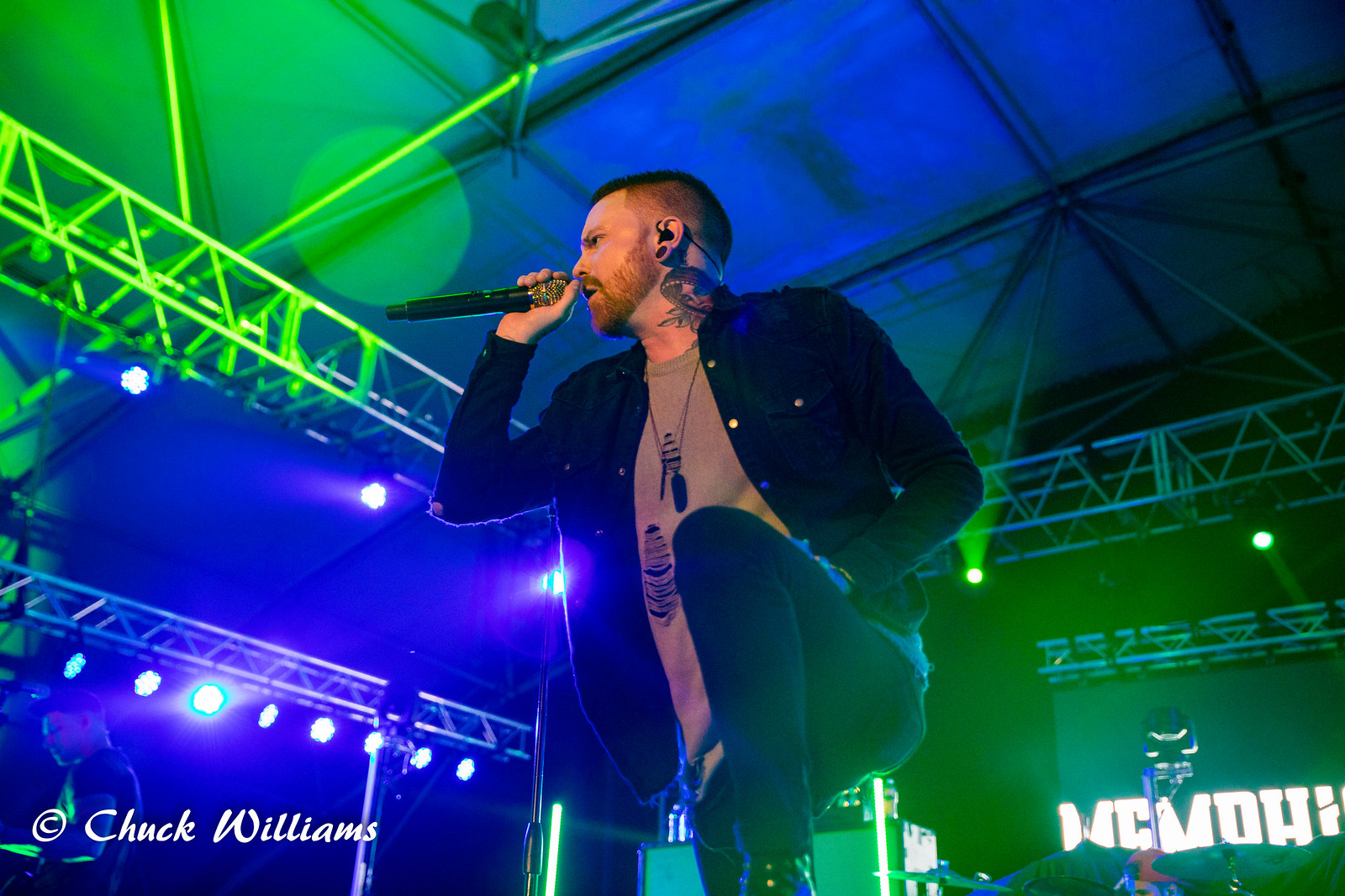The image captures a nighttime open-air concert featuring a bearded performer with a buzz cut, standing center stage. He's dressed in a black, open button-up jacket over a brown tan shirt adorned with some sort of tribal graphic or footprint decoration. He pairs this with dark blue jeans and black boots. The singer is gripping a silver-handled microphone with his right hand, holding it close to his mouth while his left leg is raised, possibly resting on a higher surface. Notably, he sports a black metallic necklace and a tattoo of a dragon or webbed creature near his left ear. The background of the stage is illuminated in blue and green hues, contributing to the vibrant atmosphere. In the lower-left corner of the photograph, a white watermark credits the image to Chuck Williams, and further to the right, illuminated white lettering suggests festival branding.